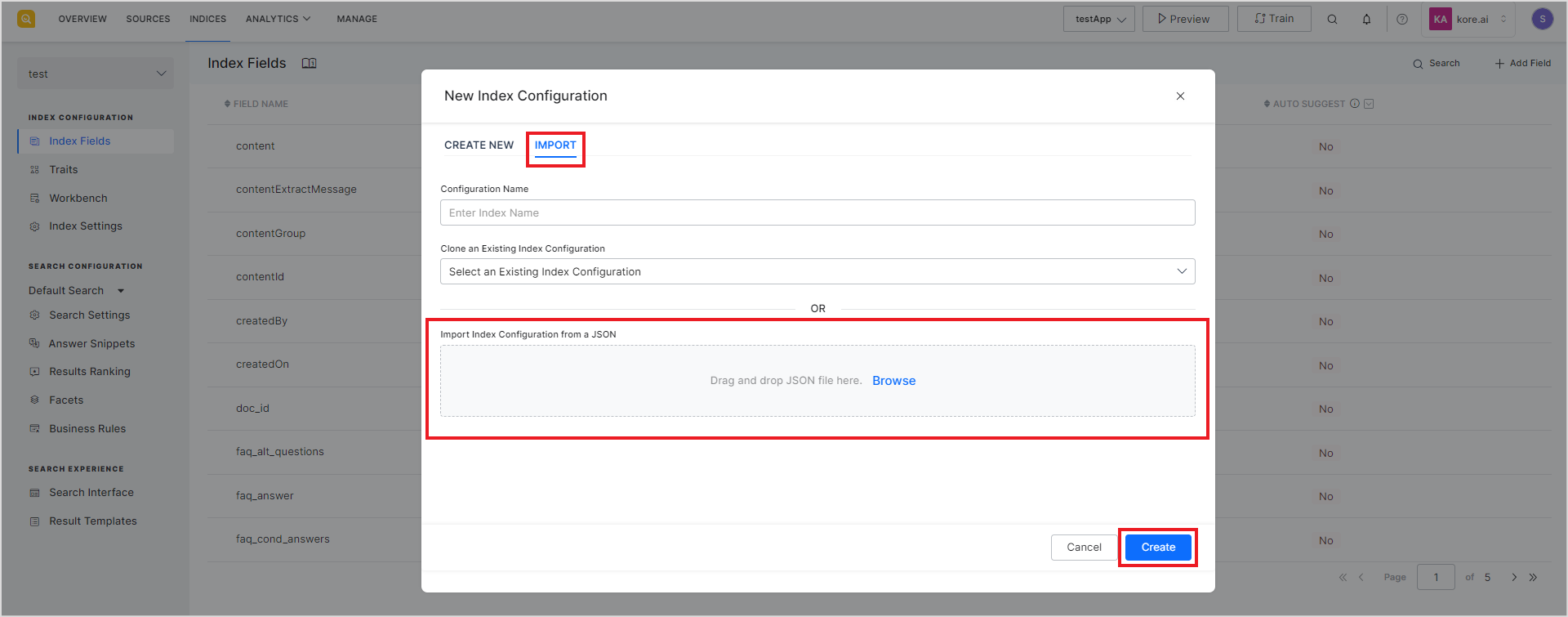A blurry screenshot depicting an admin page, possibly for a blog or content management system. The page header includes several tabs: "Overview," "Sources," "Nodes" (?), "Analytics," and "Manage," which are difficult to read. The upper right corner contains a menu, partially obscured by a grayed-out main screen. Central to the image is a pop-up titled "New Index Configuration." The pop-up offers options like "Create New" and "Import," with the latter underlined and colored blue, indicating an active state.

Within the pop-up are input fields. The first field prompts the user to "Enter Index Name," while the title of the second field is unreadable but suggests selecting an existing index configuration, featuring a drop-down menu. Another section, highlighted in red, might pertain to image settings. The bottom right corner of the pop-up contains a red-highlighted "Create" button, adjacent to a "Cancel" button. The highlighted area seems to mention importing index configuration via JSON, but the text is largely illegible.